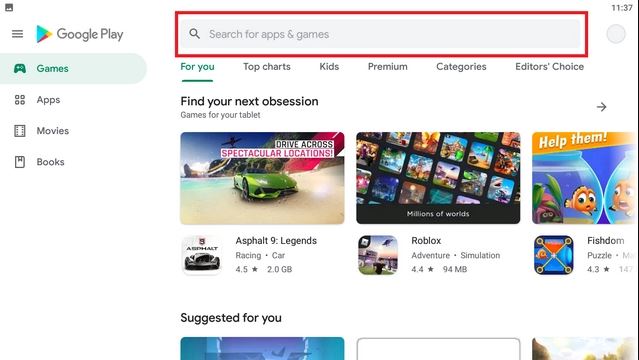This image is a screenshot of a Google Play search page displayed in landscape orientation, approximately twice as wide as it is tall. The screenshot has a thin vertical black border on the right side, with no other borders. The background is predominantly white, maintaining the typical proportions of a display seen on a computer or laptop.

At the top of the image, there is a black image icon, beneath which sits a hamburger menu featuring the Google Play icon and the text "Google Play." The Google Play icon is a distinct triangle with blue, red, and yellow colors, pointing to the right. Below this are multiple sections labeled "Games," "Apps," "Movies," and "Books," each accompanied by their respective icons. The "Games" section is highlighted with a green oval and green text.

A gray, horizontal search bar is prominently placed to the right, with a red, elongated horizontal box highlighting it. Directly below the search bar, there are options including "For You" (highlighted in green) and other categories like "Top Charts," "Kids," "Premium," "Categories," and "Editor's Choice" in black text.

The next section is headed with "Find Your Next Obsession," featuring recommendations for tablet games. There are three highlighted games: "Asphalt 9 Legends," "Roblox," and "Fishdom," each accompanied by thumbnails, ratings in stars, download size, and categories.

Towards the bottom of the screenshot is a black header reading "Suggested For You." This section includes three game thumbnails, although they are partially cut off by the edge of the screen, limiting their visibility.